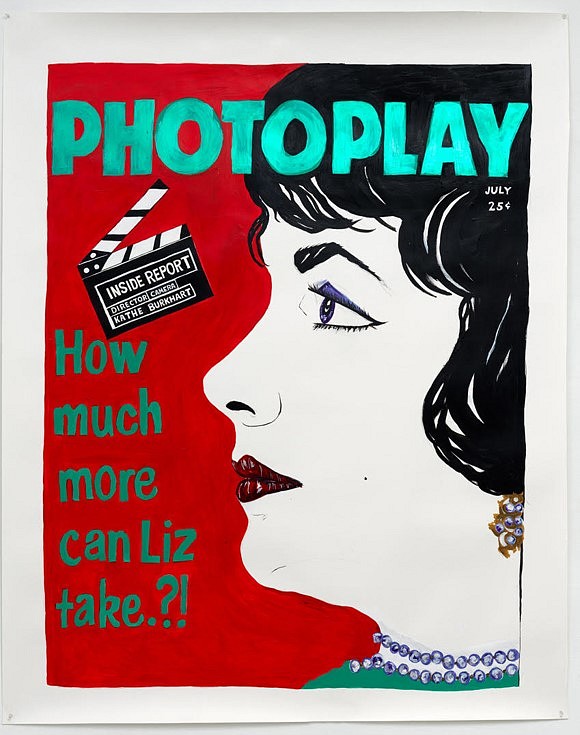The art print, hand-painted and pinned to a white wall with push pins in each corner, features a striking profile of a woman with very fair skin, dark black hair that cascades to her earrings, and dark red lipstick. Her black eyebrows frame the purplish-blue eyeliner adorning her eyes, and she wears a gold earring with blue jewels. A matching blue beaded necklace rests around her neck, complemented by her green shirt.

The background of the painting is a vivid candy apple red, which makes the subject stand out prominently. At the top of the artwork, in bold teal uppercase letters, the word "PHOTO PLAY" is displayed, and directly beneath it, in white, it reads "July 25 cents."

On the left side of the piece, there is a depiction of a clapperboard with the text "INSIDE REPORT" above it and "DIRECTOR CAMERA: Kathy Burkhardt" underneath. Below this, in dark green letters, it dramatically poses the question "HOW MUCH MORE CAN LIZ TAKE?" followed by a period, a question mark, and an exclamation point for emphasis.